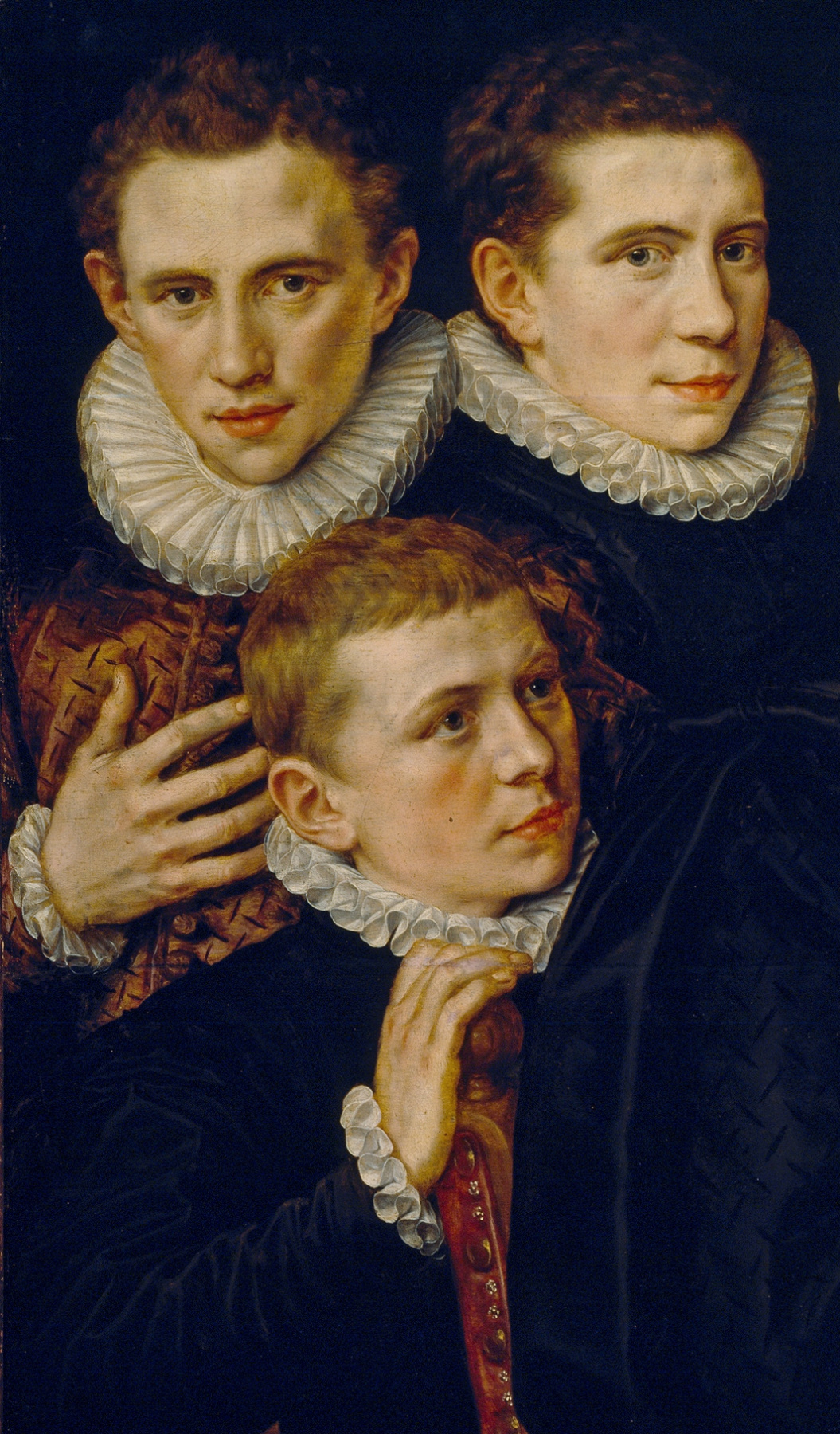This painting features a finely detailed, realistic portrait of three men, showcasing an older, Victorian-inspired style. The composition places two men at the top corners and one at the center bottom. All three wear elaborate black robes with striking, almost floral, white collars that poof out around their necks. The men exhibit distinctive, short haircuts – two with dark hair and one with red hair. The top-left man places his hand over his chest, the top-right man looks forward, and the bottom man, dressed similarly, extends his hand in front of him while looking to the right. The painting employs a rich palette that includes black, gold, brown, peach, pink, and red hues, reinforcing the elegance and presumed wealth of the subjects. The overall aesthetic and craftsmanship suggest influences from the masterful, Dutch painting techniques. This artwork, devoid of any textual elements, appears to depict possibly connected individuals, perhaps brothers, beautifully rendered in meticulous detail.